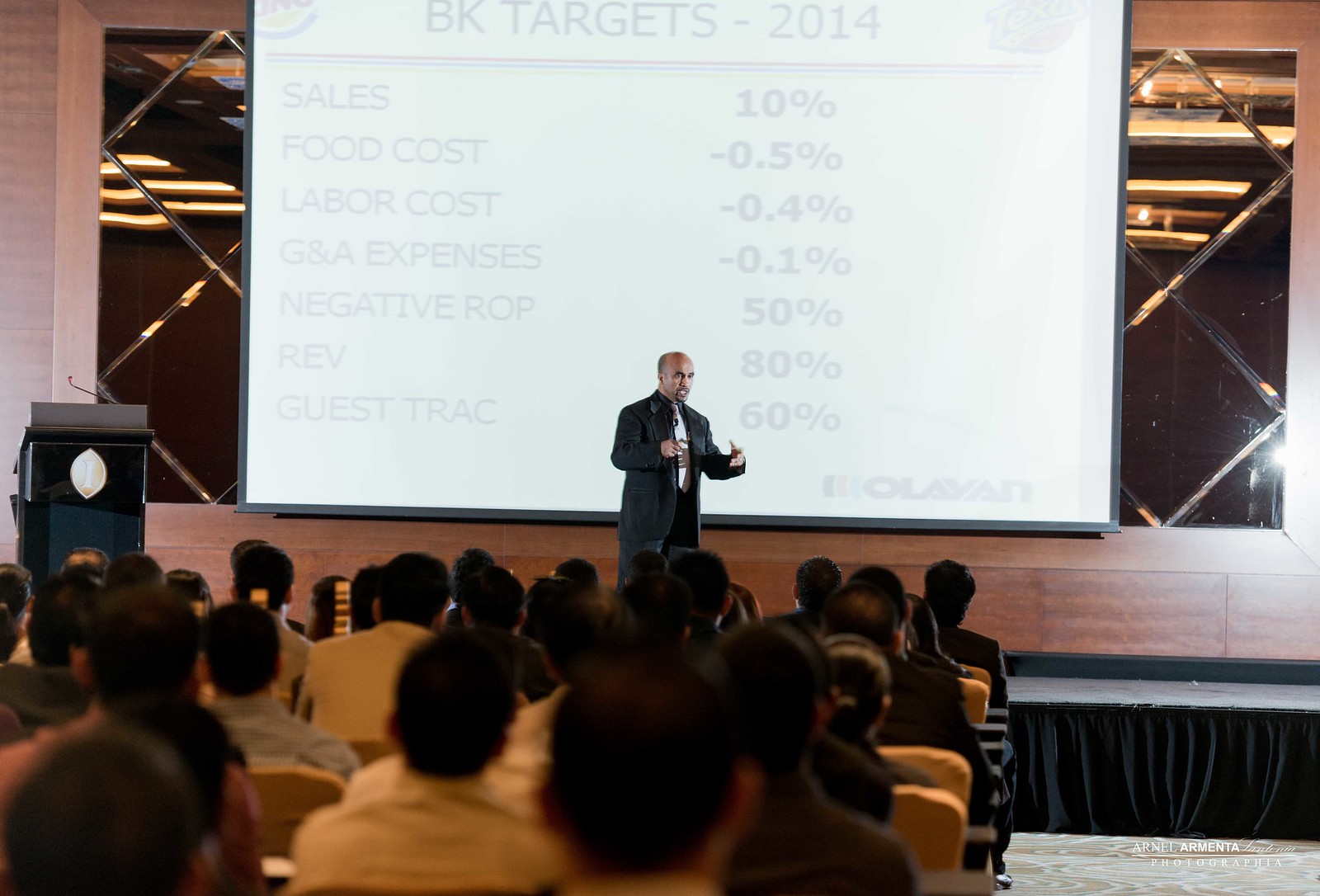This detailed caption describes a photograph of a bald man standing on a stage, delivering a presentation to an audience seated in front of him. The man, possibly of a diverse ethnic background such as black, Indian, Asian, or Latino, is wearing a black suit paired with black pants and a white tie. To his left, there is a black podium with a logo and microphone. Behind him, a very large screen, which might be mounted on a mirror-like wall, displays the heading "BK Targets 2014." Listed on the screen are various performance metrics such as sales at 10%, food costs at -0.5%, labor costs at -0.4%, G&A expenses at -0.1%, ROP at -50%, REV at 80%, and guest track at 60%. The slide also bears the name "Olyan" at the bottom and features the Burger King logo. The man is gesturing with his arms out as he speaks, engaging the audience with the data projected behind him.